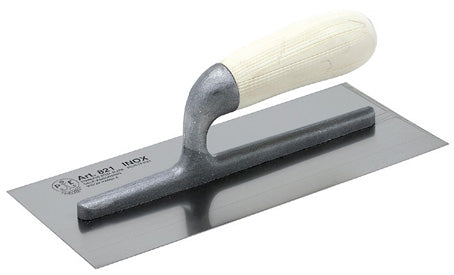The image depicts a detailed close-up of a metallic tool on a pure white background. The tool appears to be designed for smoothing surfaces, potentially used in various tasks like drywall work, carpentry, sculpting, or even art projects. It features a rectangular sheet of shiny steel, with a length of approximately 90% of the sheet being spanned by a narrow metal bar, about half an inch to an inch thick. This bar is connected to a sturdy, thick handle covered in white plastic. The flat end of the tool serves as the working surface, and the metal sheet is inscribed with "R821INOX." The overall design suggests it's a versatile instrument primarily used to spread or smooth materials, such as wet plaster, spackling compounds, or paint.